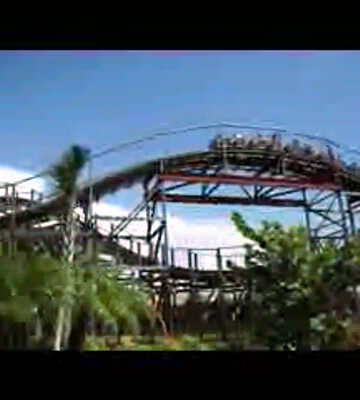This photograph captures a lively scene from a carnival ride at an unspecified theme park, possibly Disneyland, Disney World, or another amusement location. The image, measuring approximately two inches by two inches, is a low-angle shot aimed upward, presenting a viewpoint from beneath the ride. The photograph, although of poor resolution—suggesting it was taken with an older cell phone—clearly shows the roller coaster in motion, evidenced by the blurred parts that convey its speed.

Central to the photograph is the roller coaster, designed with seats hanging beneath the rail, giving the impression of passengers' feet dangling above. The ride swoops up and down along the track, with protective fencing visible behind it. The background features a bright blue sky interspersed with white clouds, indicating a sunny daytime setting. Below the ride, green foliage is visible, including pine trees with needle-like leaves and a few palm trees and shrubs, adding to the natural elements present in the theme park environment. There is no text, name, or date inscribed on the photograph.